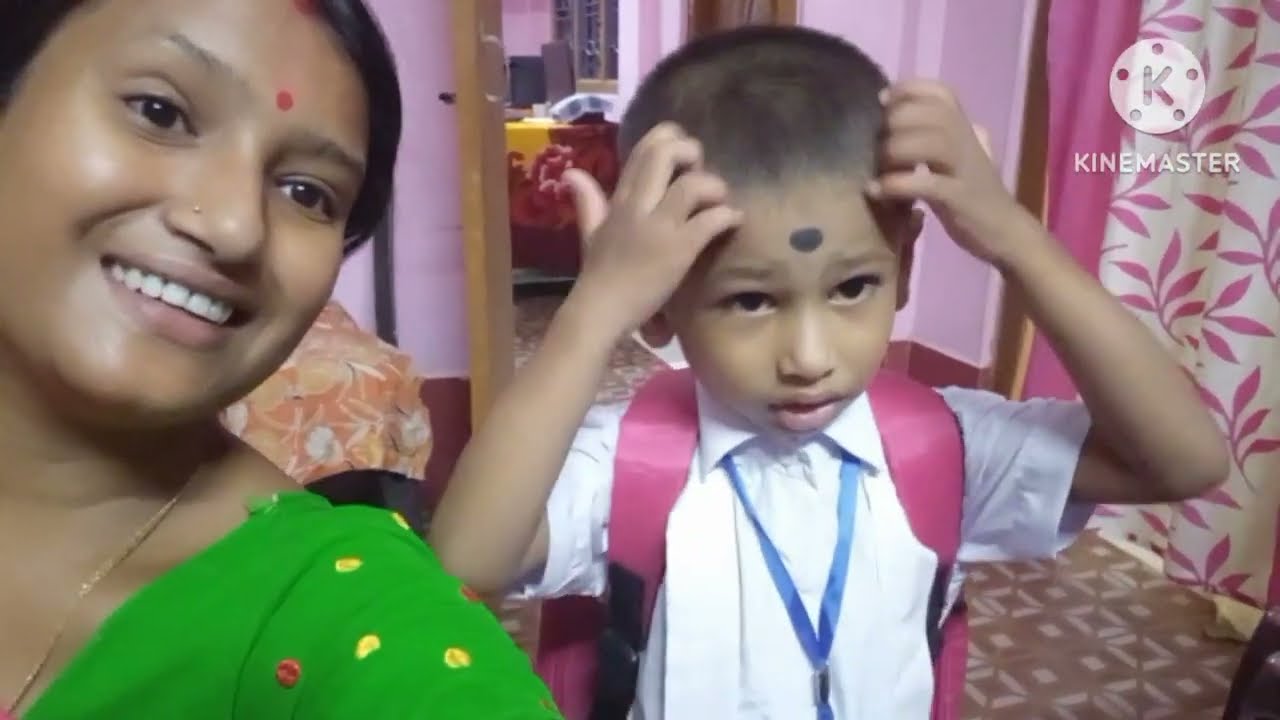The image portrays a woman and a young boy in a room with light pink walls adorned with gold borders and a gold mirror. The woman, who appears to be of Indian culture, is taking a selfie. She has a red dot on her forehead, thin black eyebrows, and black hair. She is wearing a green shirt with yellow and red spots, and a golden necklace is visible around her neck. Next to her is the boy, standing with his hands on his head, as if scratching. He has short brown hair, light brown skin, and a dark brown dot on his forehead. He is dressed in a white collared button-up shirt with a pink backpack strapped over his shoulders and a blue lanyard hanging around his neck. The room features a white curtain with pink leaves and a pink stripe, a floor with brown and white tiled designs, and an orange and yellow blanket. A brown wooden door in the background leads to another room with pink walls.